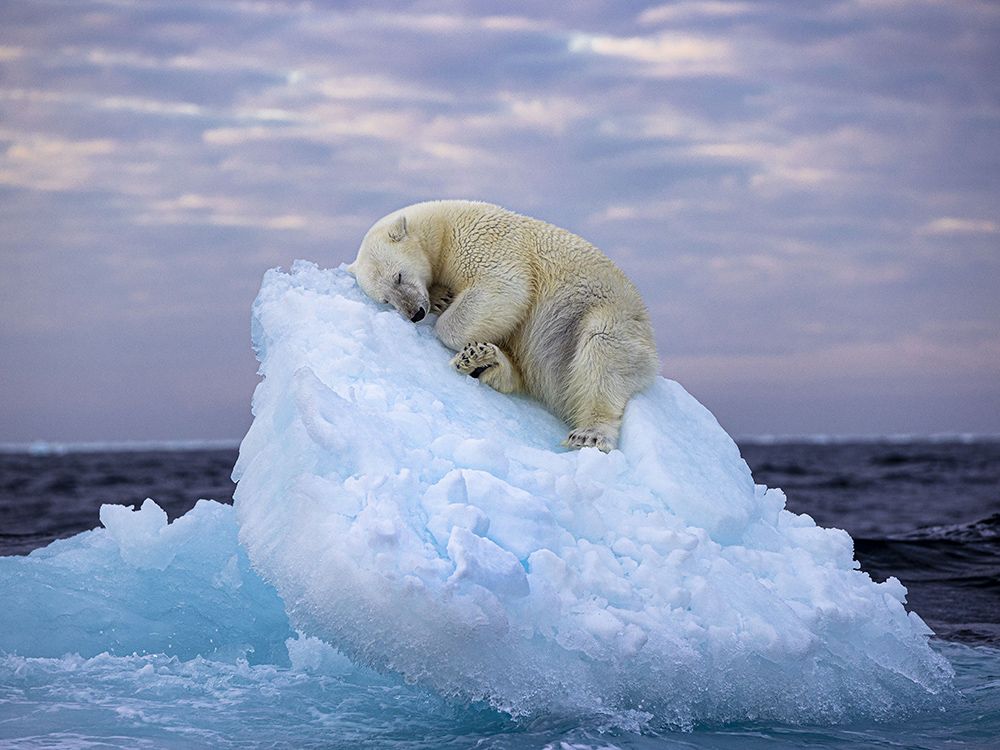This is a vivid photograph of a large polar bear sleeping on a striking aquamarine-blue glacier. The polar bear, with yellowish-white fur, is curled up comfortably, with his head and paws resting on the angled surface of the ice formation. The glacier itself extends upwards, protruding from the surrounding dark blue ocean waters, which are active and splashing against the ice. The scene is set against a backdrop of a heavily-clouded sky, tinged with hues of pink, purple, and blue, suggesting either dawn or dusk. The entire composition highlights the natural beauty and tranquility of the Arctic landscape.